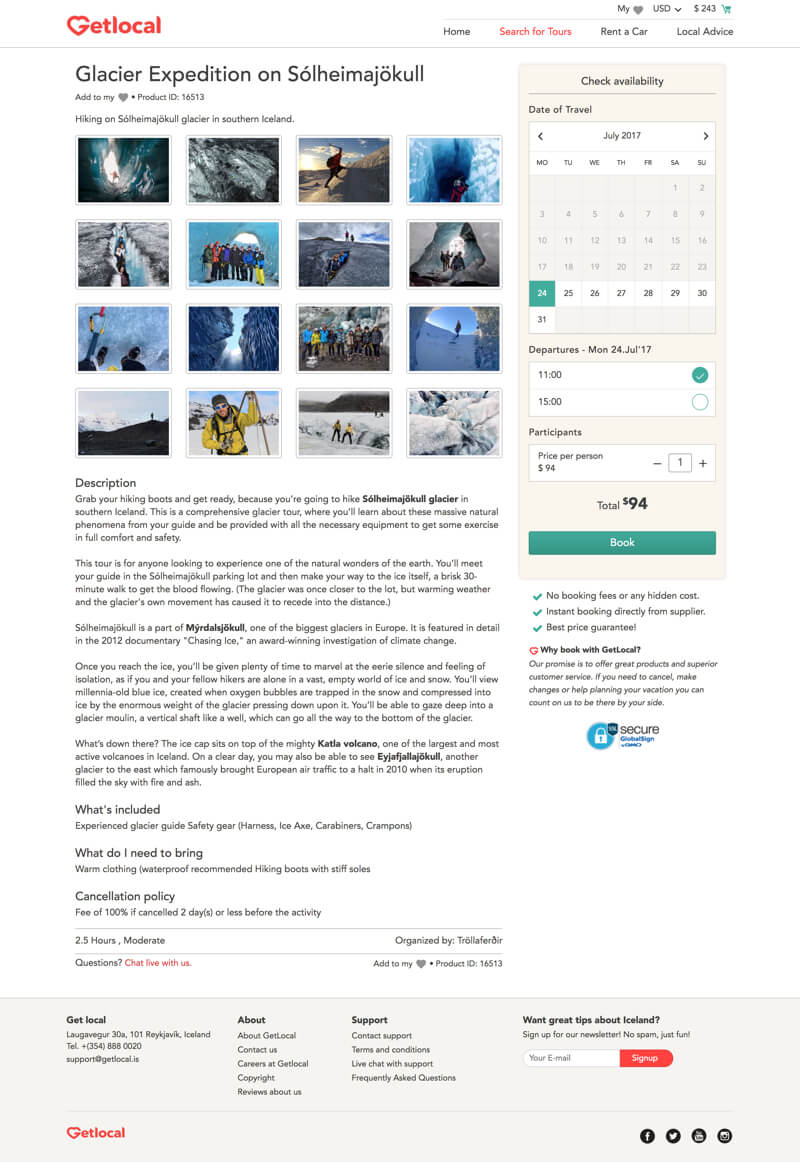Explore the majestic Solheimajokull Glacier in southern Iceland through the Get Local Glacier Expedition. This thrilling adventure invites you to hike on the Solheimajokull Glacier, known for its stunning ice formations and mesmerizing ice caves. Sitting atop the powerful Katla volcano, the glacier offers breathtaking views and a once-in-a-lifetime experience.

The expedition features detailed descriptions and captivating photos, showcasing the beauty of the glacier's icy landscape. You'll encounter extensive ice caves and group photo opportunities, with some images highlighting the solitude of a single explorer amidst the vast ice fields.

The adventure is rated as a moderate difficulty level and takes approximately two and a half hours to complete. Booking is straightforward: you can select your preferred date and time using the on-site calendar, and the total cost for this unforgettable experience is $94. Secure your spot today by clicking the 'Book' button and get ready to embark on an exhilarating journey through the icy wonderland of Solheimajokull Glacier. Cancellation policy details are available at the bottom of the page.